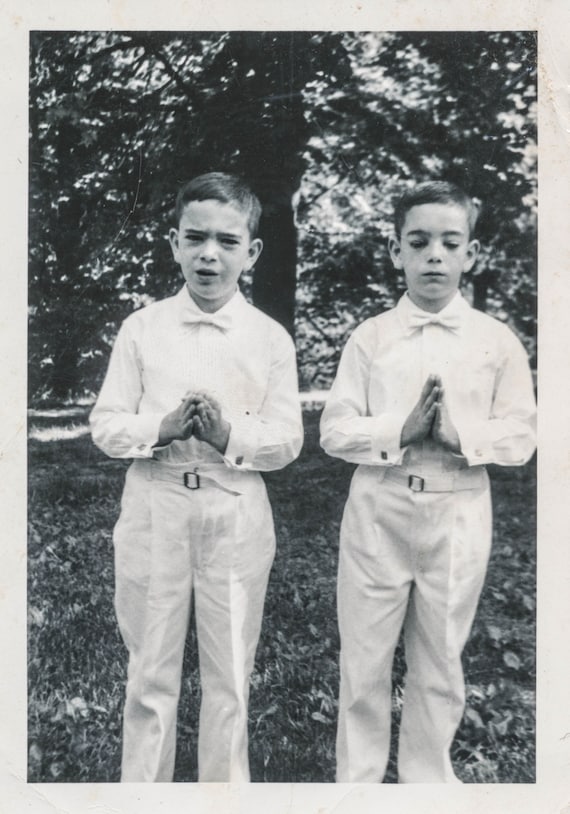The image is an old black and white photograph, likely from the 1950s or 60s, featuring two twin boys standing side by side on a grassy area scattered with leaves, in front of large trees that dominate the background. Both boys are dressed in identical, old-fashioned Sunday church attire, consisting of white shirts, bowties, pants, and belts. They have a solemn demeanor, with their hands folded together in a gesture resembling prayer. The boy on the left has his eyes open and appears somewhat sad, gazing directly into the camera, while the boy on the right has his eyes closed, maintaining a calm and serene expression. The photograph has an old-fashioned white frame around it, reinforcing its vintage aesthetic.